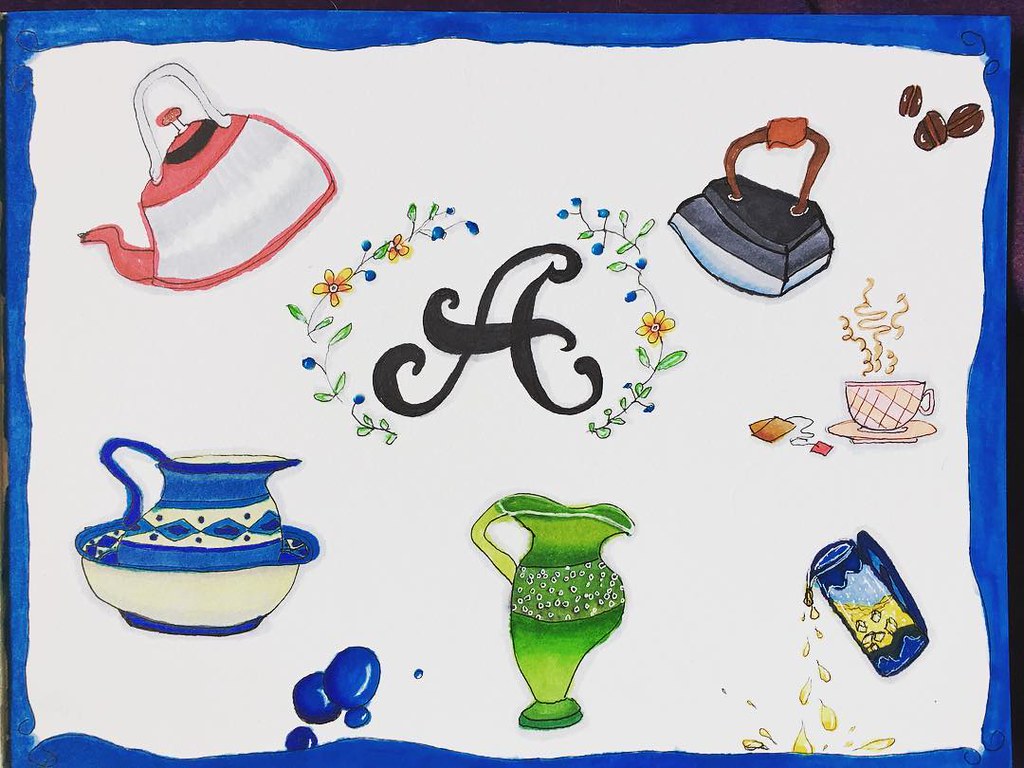The drawing is an intricate still life composition featuring an assortment of household items and natural elements. At the heart of the image is a large, decorative cursive letter 'A,' elegantly positioned amidst a cluster of entwined stems and leaves. Surrounding this central element, there are gracefully sketched teapots, kettles, and vases, each detail meticulously rendered. In the top right corner of the artwork, a handful of coffee beans and a steaming teacup filled with coffee add a cozy touch to the scene. The entire piece exudes a sense of charm and careful craftsmanship.